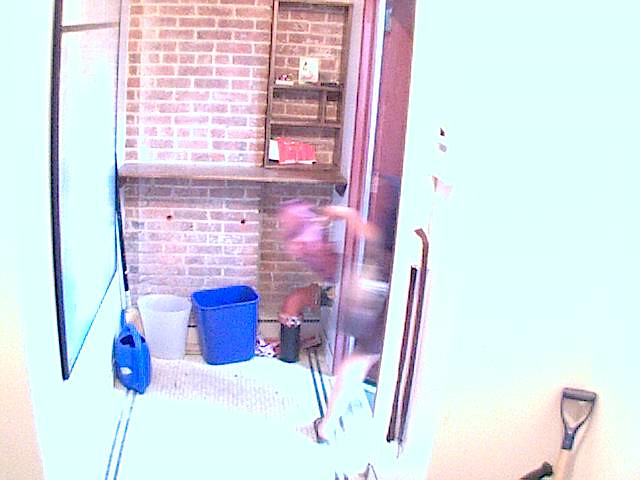The photograph captures the interior of a bright indoor space, where the light exposure gives it a washed-out appearance. Centrally, a faded red brick wall stands out at the end of what appears to be a hallway or an alley. Attached to this brick wall is a wooden shelving unit and a partial wooden desk or divider. To the left of the brick wall, there might be a glass window. At the bottom of the image, a blue recycling bin and a smaller white trash can are positioned. On the right side of the image, there's a blurry figure, indicating someone is in the process of entering or exiting through a door. Additionally, the bottom right corner features a shovel, propped against a white wall above a section of white carpet. The overall brightness of the scene suggests it's a strongly illuminated indoor area.